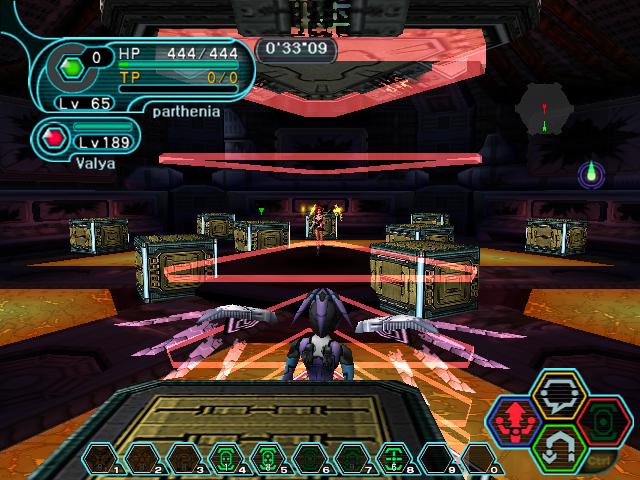The image is a pixelated screenshot from an old-fashioned video game, reminiscent of titles from the Sega Dreamcast or original PlayStation era, suggesting it's not the latest technology and has lower-resolution graphics. The scene is dark and colorful, with red, blue, black, gold, and purple hues dominating the palette.

In the foreground, there's a distinctive alien-like robotic creature, characterized by a purple goat-like appearance with long, downward-pointing ears. This figure stands near a table setup. Two types of crafts, potentially flying towards this robotic figure, flit on either side of it. On the floor, there are lit-up, yellow square shapes, resembling a grid or pathway, and several blue treasure chest-like boxes edged with white lines, all closed.

Above, a series of triangles hover in alignment: a red and pink triangle at the top, a thin one hanging in the air below it, and another pink triangle with yellow accents on the floor. At the top of the screen is a scoreboard displaying various game stats: HP 444/444, TP 0/0, LV 65, and LV 189, accompanied by the names "Parthenia" and "Valya." The timer reads 0:33:09, indicating an elapsed time. 

In the distant background stands a scantily clad female figure, illuminated faintly by lights but too far away to discern her facial features. The immersive, battle-ready environment suggests the game scenario likely involves confronting this figure.